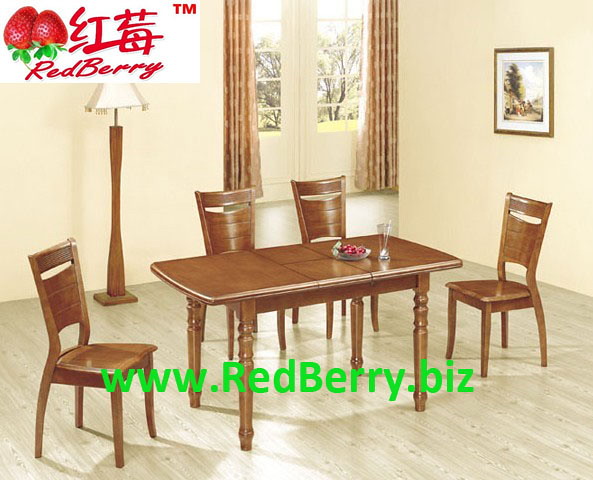The image depicts a stylish dining room set up, seemingly arranged for a furniture advertisement. Prominently displayed is a large wooden dining table centered in the shot, featuring a three-panel design with a distinct arrangement: the middle panel is a narrow rectangle, flanked by square panels on either side. On the table rests a small bowl and a single glass, adding a touch of realism to the setting. Surrounding the table are four well-crafted wooden chairs—two positioned along the longer side and two more partially visible at the ends.

The room exudes a warm ambiance, with beige walls and wooden flooring lending a cozy atmosphere. Hanging on the right wall is a picture of a tree, complementing the earthy tones of the room. To the left, there is a wooden lamp with a white cover, providing soft illumination. The space is framed by brown curtains draped over French windows, offering a glimpse of an inviting outdoor scene with large trees visible through the glass.

Branding elements are prominently featured in the image: the top left corner showcases the RedBerry logo, which includes two upside-down strawberries forming a heart shape, with green stems still attached. Accompanying the logo are Chinese characters representing the brand name and a trademark symbol. Additionally, a green watermark with the website "www.redberry.biz" runs across the lower part of the image, reinforcing the brand's identity and online presence.